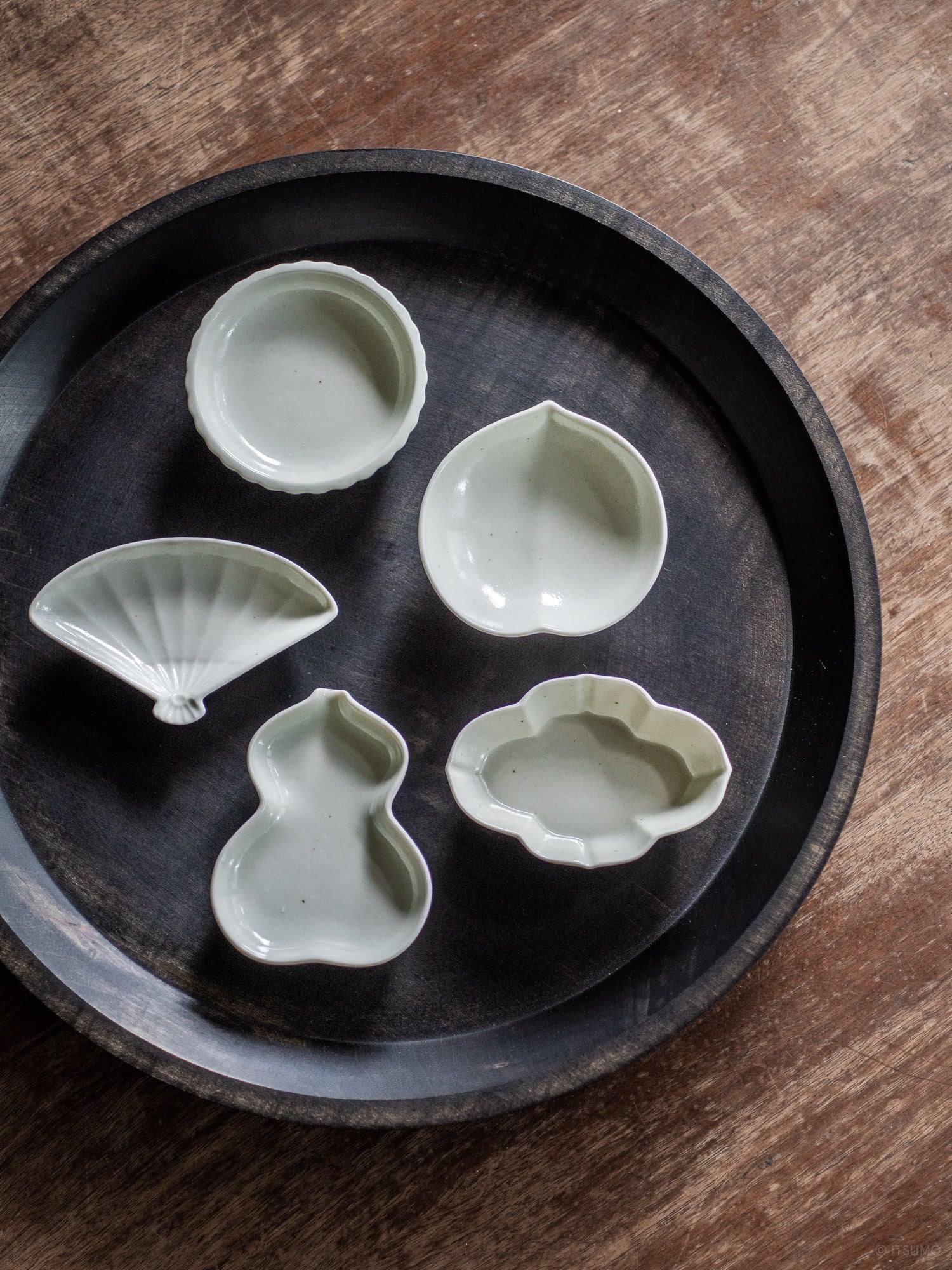This image shows a worn brown wooden table with a dark circular tray or bowl placed on it. The tray, which resembles a pie pan, contains five distinct white objects that appear to be molds for shaping materials. These molds include a seashell, a snowman, two circles, and one that resembles a clover or an oriental fan. The detailed mold shapes can be used for creating various designs, with the circular tray’s edges slightly jutting upwards, giving the arrangement a structured appearance.